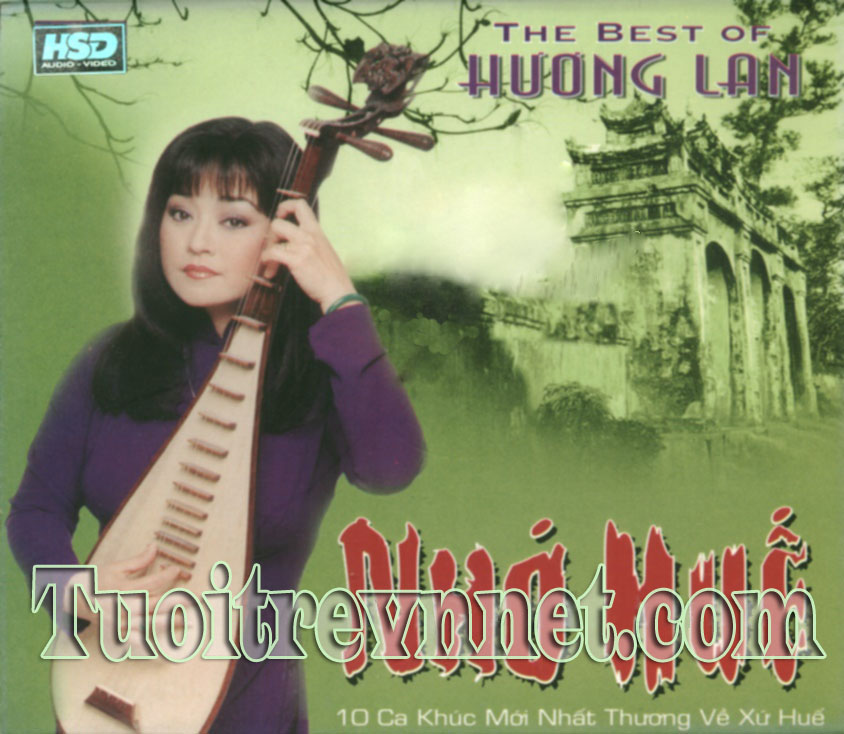The image appears to be a scan of a music album cover featuring an East Asian aesthetic. Dominating the left side of the image is a photograph of a woman with long, dark hair, clad in a purple long-sleeved dress, holding a long, brown, stringed instrument – possibly a sitar or lute-like instrument. The background is primarily green, with an intricate sketch of stone arches and gateways, suggestive of a castle, in the upper right corner. There's also a mix of sepia tones with branches and leaves touching the top of the image. In the upper left corner, the logo "HSD" is prominently displayed, while in the upper right, the title "The Best of Huang Lan" is written in purple text. Towards the bottom, red text overlaying white, transparent text reads "tuotrevenet.com", along with what appears to be additional details in Vietnamese, "10-ca khuc moi nhat thuong ve xu Hue." The overall scene is one of serene grace, tying together traditional music and historic architecture.